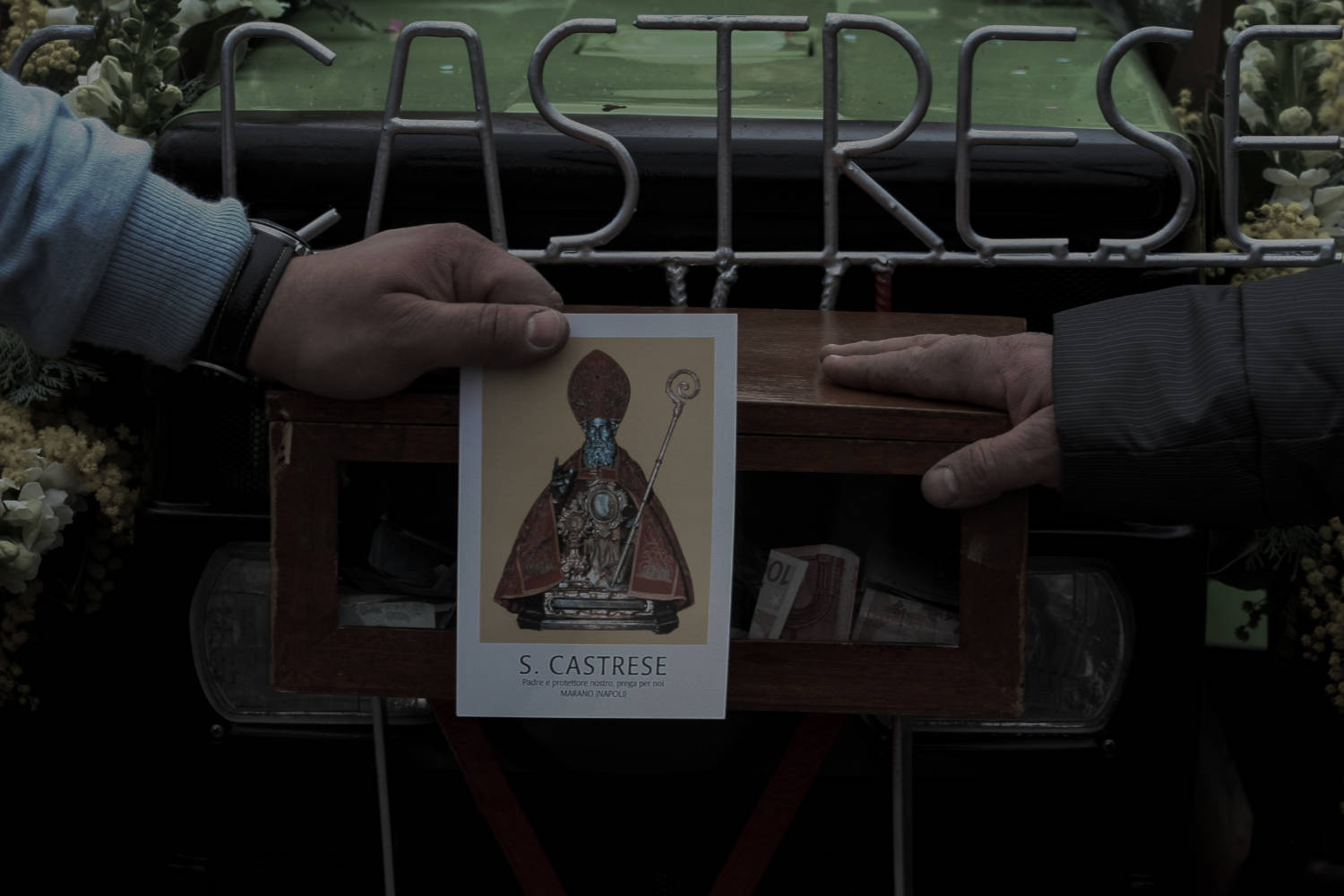The image features a wooden donation box positioned at the center, with a clear front panel revealing various bills inside. Surrounding the box are white flowers, and it is flanked by two hands. The left hand belongs to a person wearing a gray sweater and a watch with a brown strap, and they are holding a card depicting a saint with the inscription "S. Castrese." The right hand rests openly on the box and is clad in a black jacket with white stripes. Behind the box, metallic letters spell out "Castrese," hinting at the setting being a church or religious site. In the backdrop, there are indistinct objects that resemble headlights, adding a mysterious element to the scene.